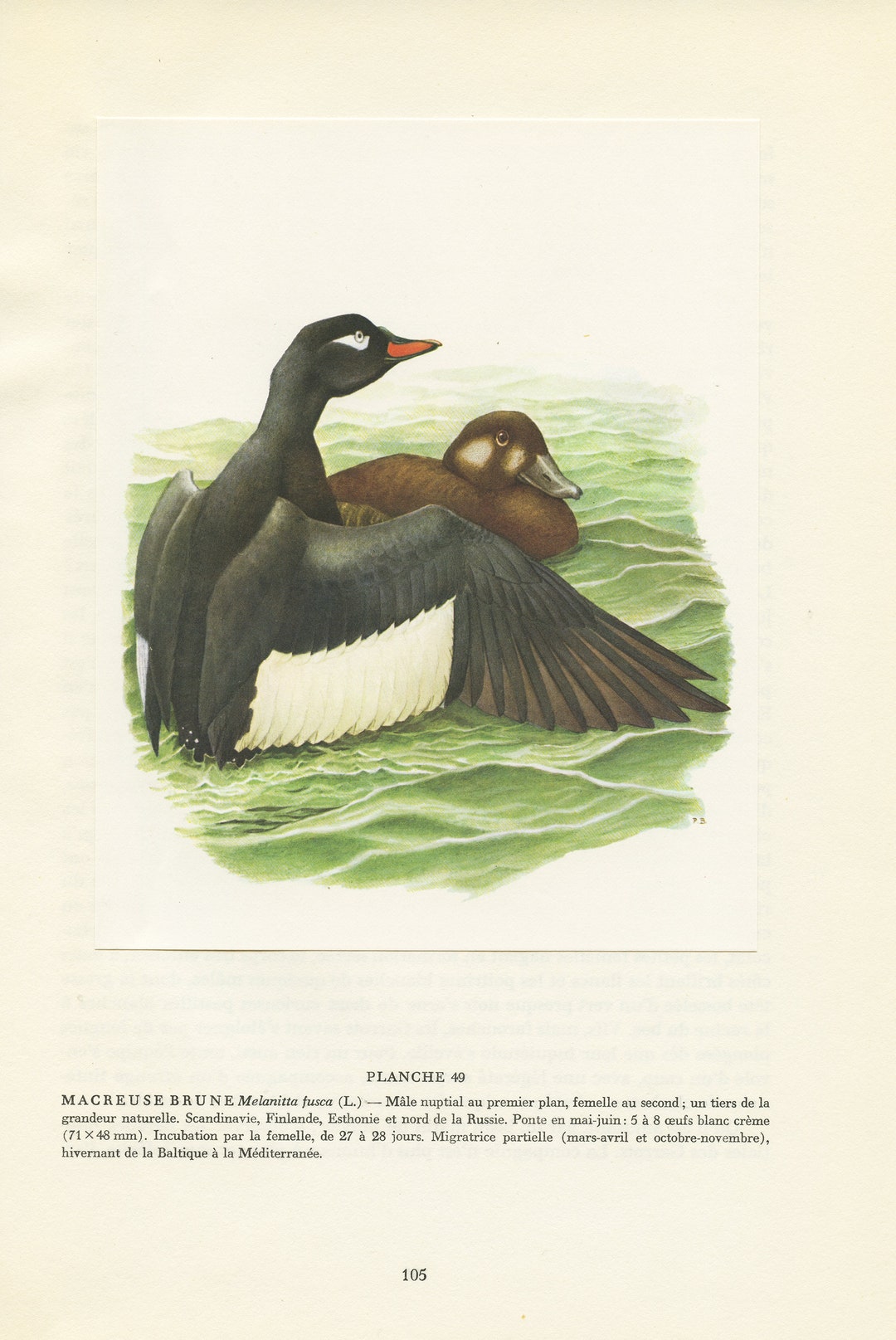This illustration, reminiscent of vintage birdwatching books with its off-white, slightly yellowed pages, appears to be a watercolor originally, later reproduced for publication. It features two birds in a water habitat, depicted with greenish, slightly wavy water. The foreground showcases a striking black and white duck, its orange beak and partially outspread wings suggesting dynamic movement. Noticeable details include white feathers around its eyes and wings. To the right, a smaller brown duck, likely the female, is swimming calmly. Beneath the illustration, French text explains their species and habitat, identifying the page as 105 and mentioning "planche 49." The overall scene emphasizes traditional bird species documentation, typically highlighting male and female pairs in their natural habitats.